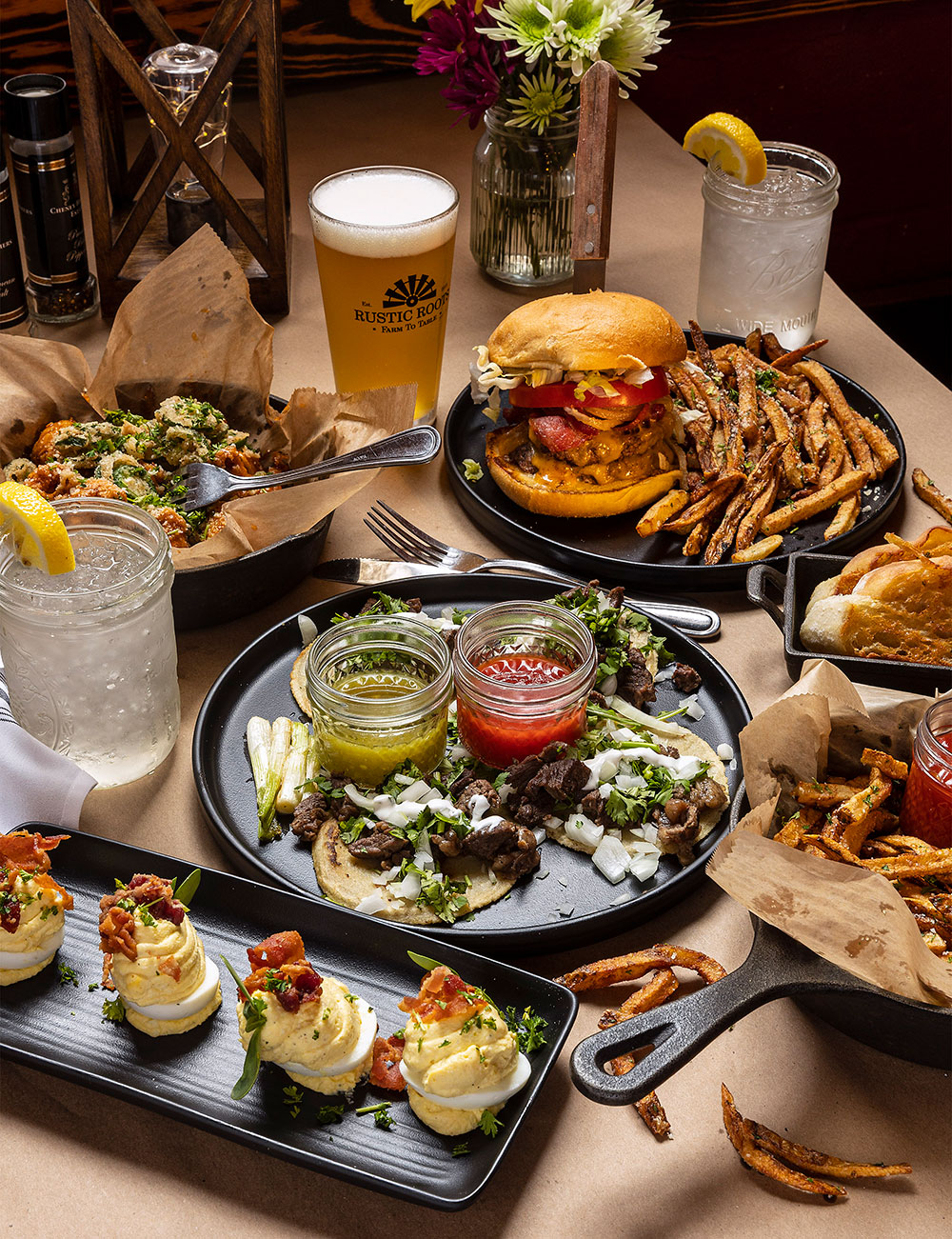The image depicts a richly adorned restaurant table filled with a variety of dishes and beverages. At the top left corner, a basket contains a breaded meal with a fork stuck in it, suggesting it's ready to be eaten. Moving to the right, a large hamburger is accompanied by a generous serving of French fries layered throughout, garnished with parsley and sprinkled with white cheese. Above this meal, a mason jar filled with ice water and a slice of lemon adds a refreshing touch, mirrored by another similar mason jar towards the center-left of the image. Sitting beside it is a glass of amber beer, likely in a glass marked "rustic rooms," hinting at the venue's quaint, homey atmosphere.

Central to the spread is a black tray showcasing five tacos adorned with onions and celery, complemented by two vibrant dips—one green, one red. Scattered around the table are more items, including a basket of fries on the right and a skillet holding additional fries and possibly bread in a loaf pan. In the foreground, a rectangular dish displays an intriguing appetizer, possibly deviled eggs or a fluffy, whipped potato concoction with bits of bacon on top. The backdrop reveals a touch of ambiance with a lantern-like structure holding an Edison bulb and a clear jar partially brimming with colorful flowers, adding a cozy yet elegant vibe to the dining experience. All the food is presented on black, cast iron-like tableware, adding a rustic charm to the culinary display.